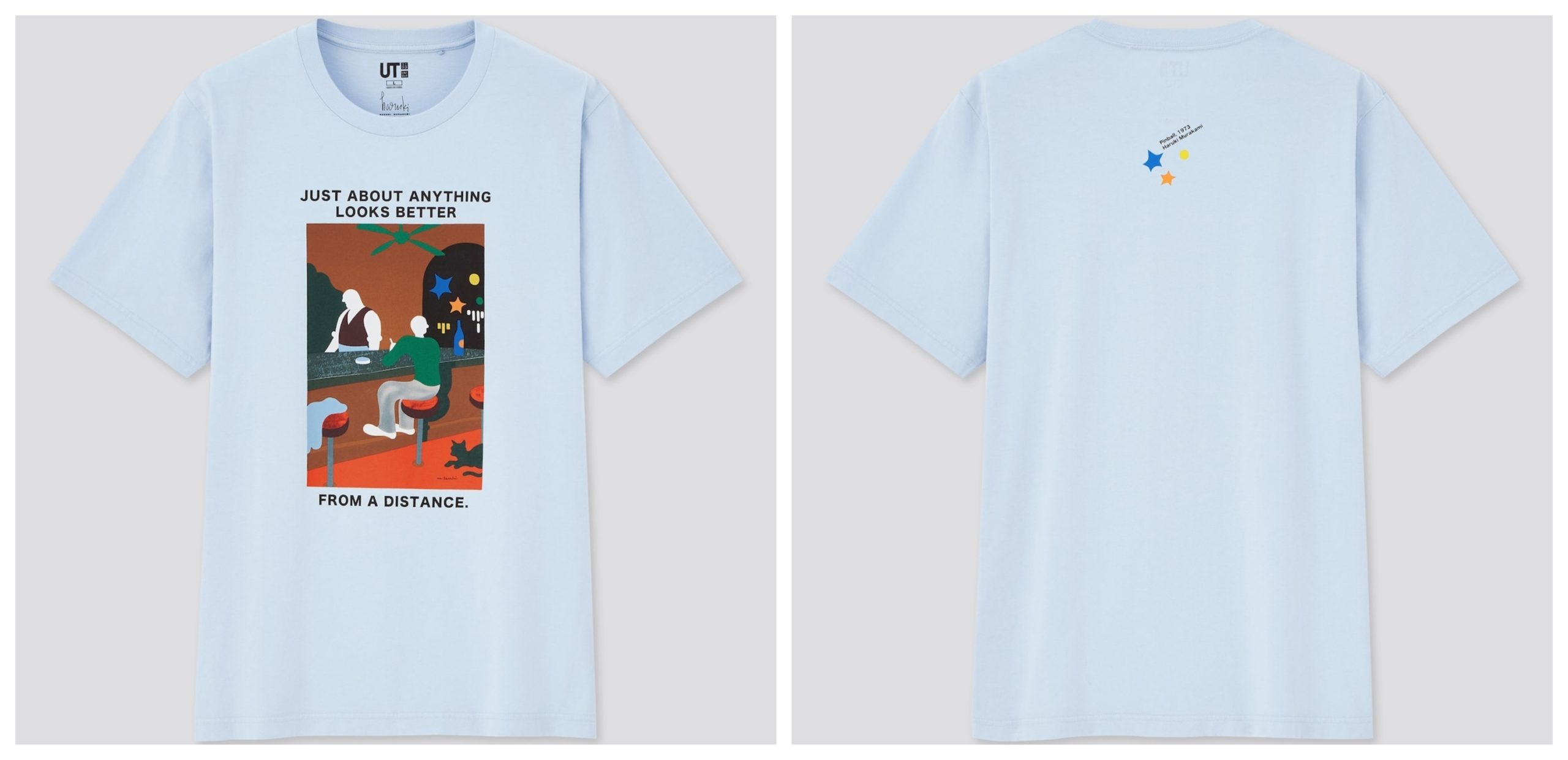The image features two photos placed side-by-side, each showcasing a light blue, short-sleeve t-shirt. The photos are set against a gray background and are separated by a white line, creating a distinct space between them. The left-hand photo displays the front of the t-shirt, characterized by a cartoon image of a person sitting on a red-topped bar stool. The person, viewed from behind, gazes to their right. Behind the bar, a bartender, facing left, attends to duties. Above this illustration, the text reads, "Just about anything looks better," while below it, the phrase completes with, "from a distance." The right-hand photo reveals the back of the t-shirt, maintaining the same clean, light blue appearance.